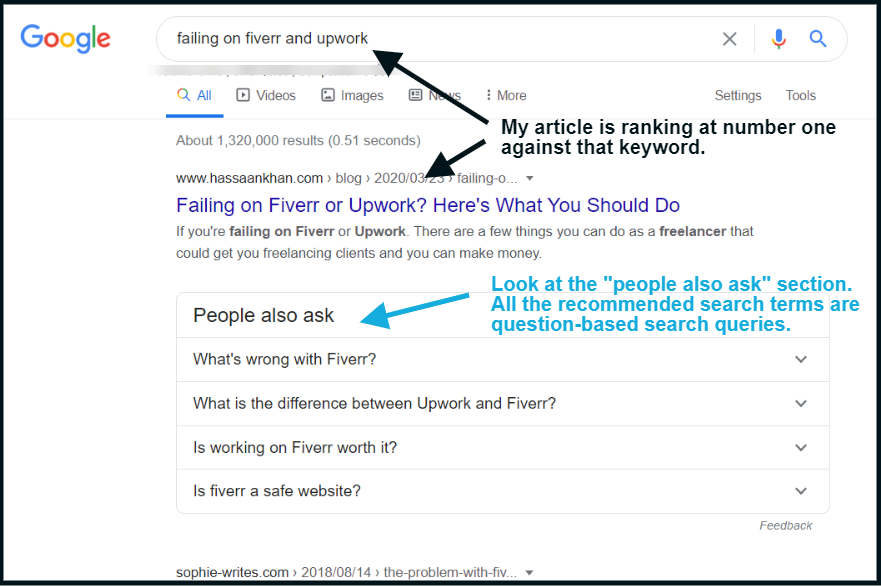A Google search for "failing on Fiverr and Upwork" is displayed, showing the primary link titled "Failing on Fiverr, Upwork? Here's What You Should Do." This link is highlighted with an arrow pointing to it. The snippet beneath the link provides a brief overview, mentioning that freelancers can take certain steps to secure clients and generate income if they are struggling on these platforms.

Fiverr and Upwork are described as websites where freelancers and self-employed professionals offer their services, which can then be hired by clients as needed. Alongside the primary search result, Google's "People also ask" section is shown with questions such as "What's wrong with Fiverr?" "What's the difference between Upwork and Fiverr?" "Is working on Fiverr worth it?" and "Is Fiverr a safe website?" An additional highlighted section reveals part of a link from sophie-writes.com, indicating an article published in 2018.

Arrows are also drawn to the search bar and the first search result, with a caption noting, "My article is ranking at number one against that keyword." The detailed annotations emphasize the result's significance and the relevance of the article to freelancers seeking advice on these platforms.